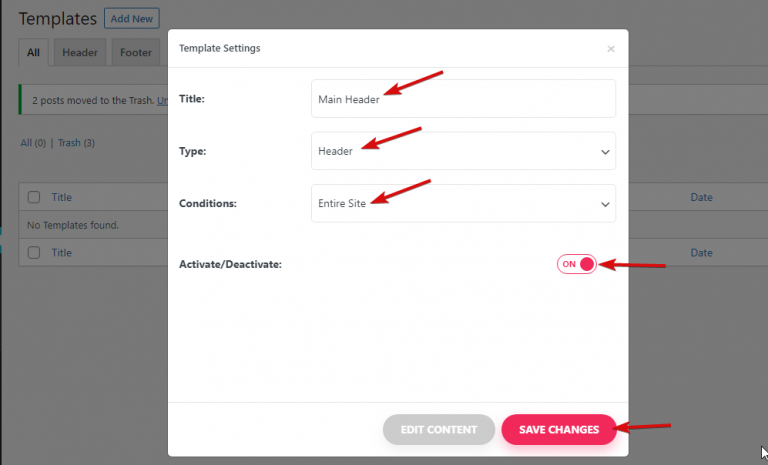The image depicts a settings page for customizing a website template. At the center of the page, there's a prominent white dialog box titled "Template Settings" in grey text. This dialog features several options, each highlighted with red instructional arrows. 

The first option, labeled "Title" in bold, includes a text box containing the phrase "Main Header," with a red arrow pointing to it.

The second option, "Type," also in bold, features a selectable item marked "Header," indicated by another red arrow. Adjacent to this option is a grey, downward-facing arrow, suggesting that the header style can be changed.

The third option, labeled "Conditions," includes the phrase "Entire Site," with a red arrow pointing to it. This box also has a grey downward-facing arrow, implying additional conditions can be selected.

Additionally, there is an "Activate/Deactivate" toggle switch, shown in the on position, which is also marked by a red arrow.

At the bottom of the dialog box, there are two buttons: "Edit Content" and "Save Changes," with the latter being indicated by a red arrow. 

The arrows likely serve an instructional purpose, guiding users through the various features available. The backdrop of this central settings box reveals a broader templates management page, with options listed such as "All," "Header," and "Footer," indicating that this is a comprehensive interface for website customization.